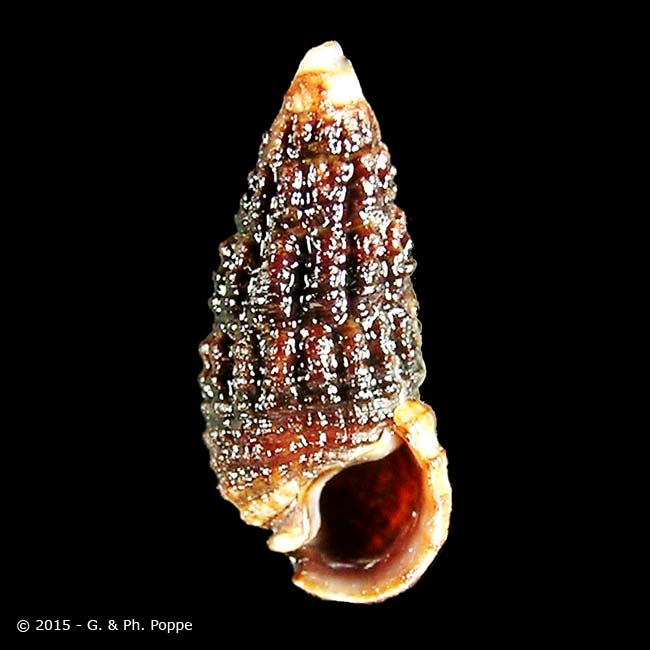This image features a meticulously adorned, tall cone-shaped snail shell, showcased upright against a plain black background, drawing full attention to its details. The shell, predominantly light brown and white, is embellished with glossy red and brown paint, giving it a glamorous appearance. The tip and the area around the opening exhibit golden and yellow hues, transitioning to a deep reddish-black within the hollow interior. The texture of the shell is characterized by horizontal rings and numerous small divots, possibly a result of natural formation or erosion. Positioned centrally in the frame, the shell's wider base curves into an opening at the bottom. In the bottom left corner, the image features a small white text copyright notice, reading "© 2015-G.&PH.POPE."